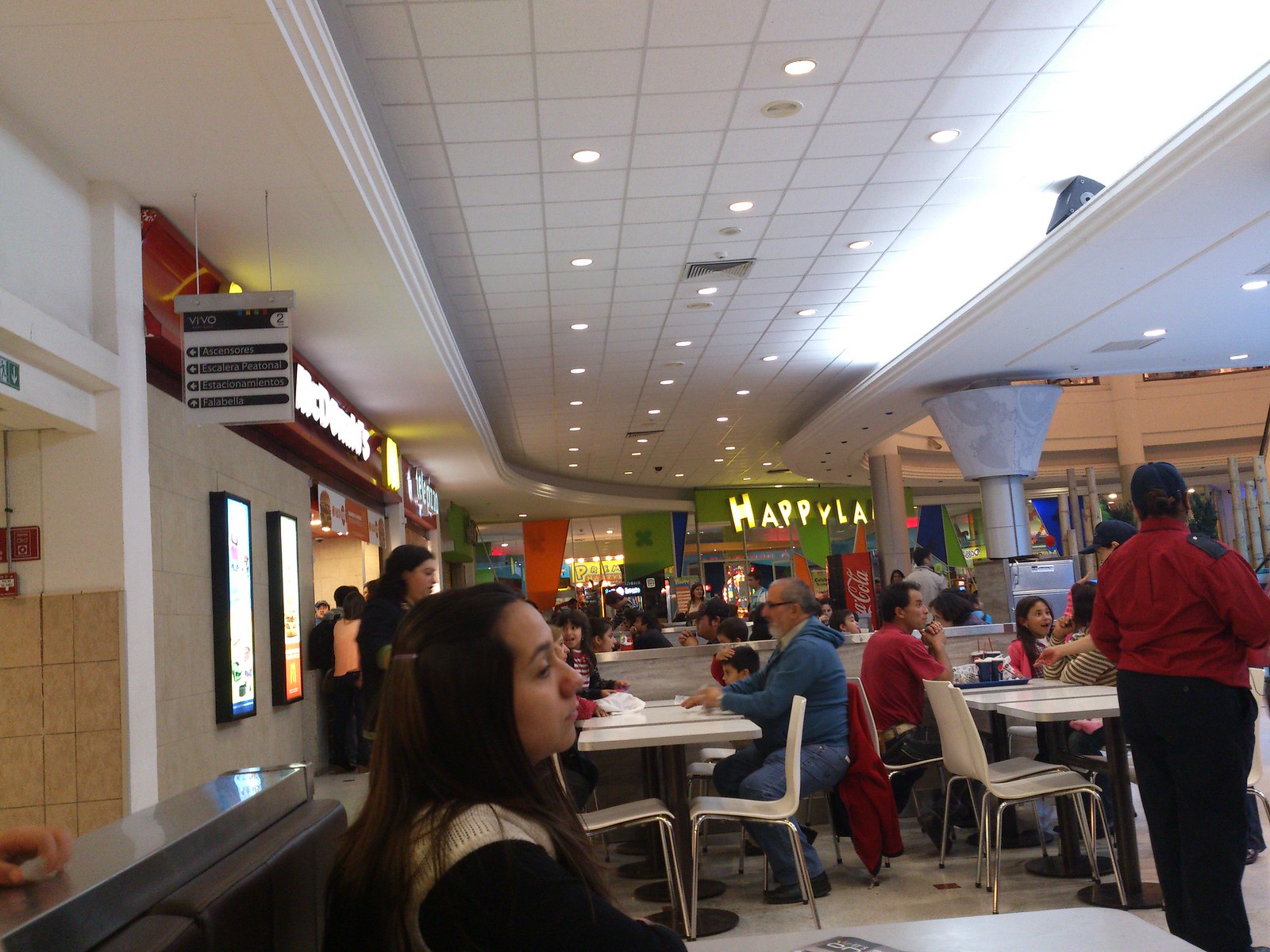This photograph captures a bustling indoor food court, likely situated in a shopping mall, with a variety of comfort and fast-food options. The scene is anchored by a prominent McDonald’s on the left side, with its recognizable logo clearly visible. Adjacent to McDonald's is a Telepizza outlet. In the background, the bright yellow letters of "Happyland" are partially visible on a green wall, suggesting a nearby children's amusement area adorned with Pokémon prizes. The ceiling of the food court is white with numerous spotlights providing ample lighting.

In the foreground, a woman in a black dress with a white coat over it is seen from the side, sitting at one of the many white tables scattered throughout the area. Near her, to the right, stands another woman in a red long-sleeve shirt and black pants. Further into the food court, a man, possibly in his 60s with longer hair, a white beard, wearing glasses, and dressed in jeans with a blue top, is seated and engaged in conversation with a woman dressed in black across from him. The vibrant and lively atmosphere is complemented by the presence of a Coca-Cola machine in the distance, adding to the overall lively and busy ambiance of the food court.